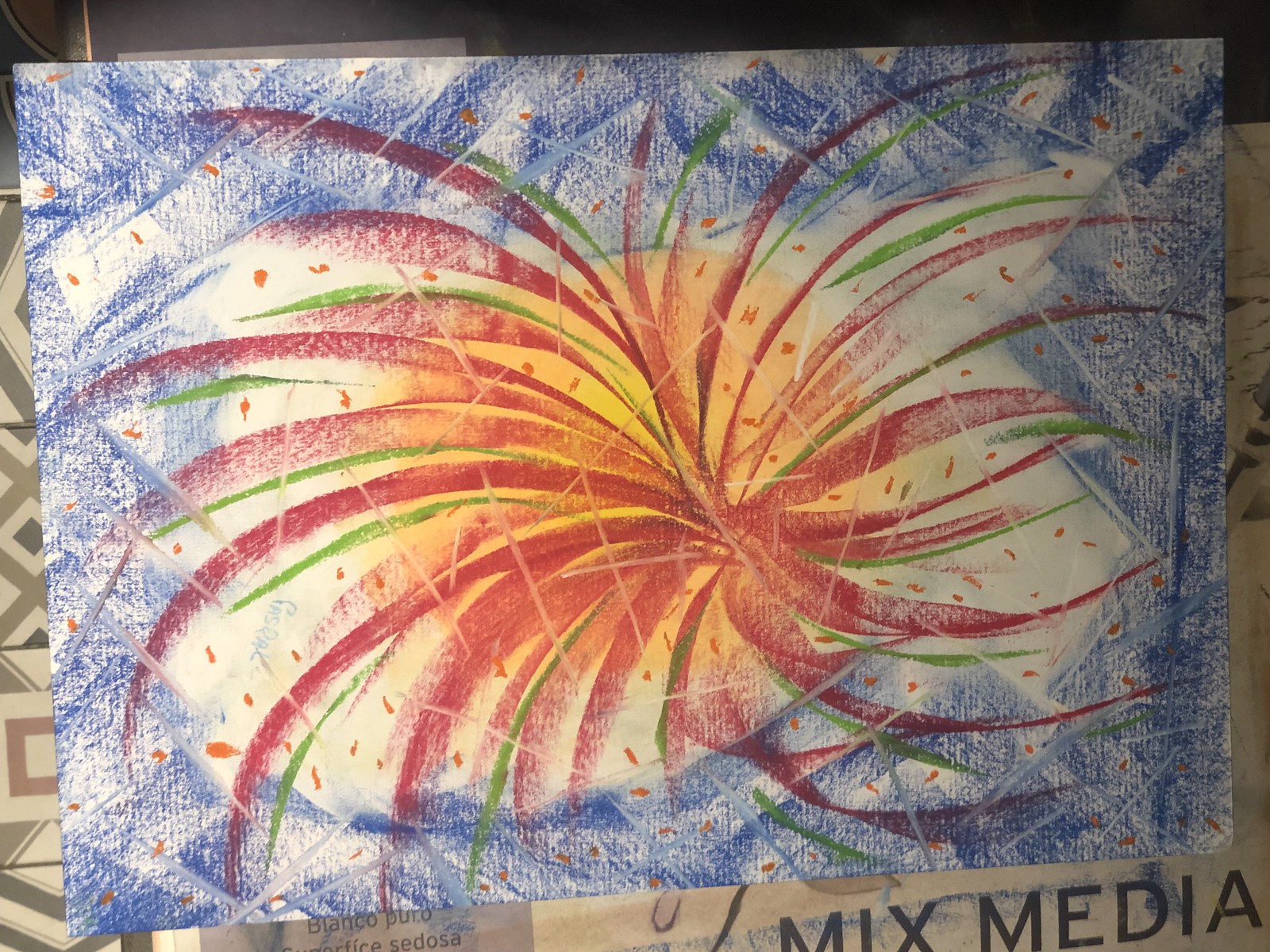The image depicts a vibrant mixed media artwork created with crayon, showcased on a tiled floor. The artwork, presented on a piece of thick, textured paper, stands out with a captivating design at its center. Dominated by a blue and white clouded sky background, the scene features a prominent glowing yellow sun that radiates warmth. At the heart of the composition, a striking burst resembling a spiky flower or fireworks display is illustrated with a dynamic mix of red, blue, and yellow hues. Red firework-like lines and red specks resembling confetti spread outward from the center, adding a sense of celebration and energy. The border of the artwork is highlighted with crisscross patterns in blue and white. On the bottom right corner of the tile floor is a magazine page with the words "mixed media," hinting at the artwork's diverse creative influences.